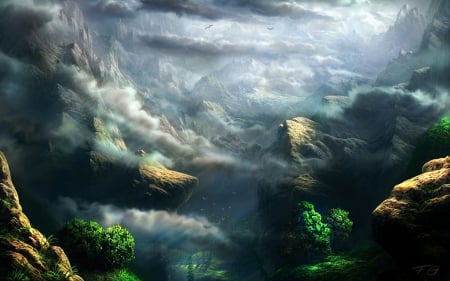The painting presents a fantastical landscape dominated by an ominous, dark bluish-gray sky filled with textural, distinct clouds. Thick white and green mists envelop the towering, sharp rock formations that frame a lush valley. The valley, positioned at the bottom center of the painting, is populated with green grass and trees. These rock formations ascend steeply, creating a cup-like enclosure around the valley. Birds can be seen soaring through the thick, gray clouds, adding a dynamic element to the otherwise serene and mystical scene.